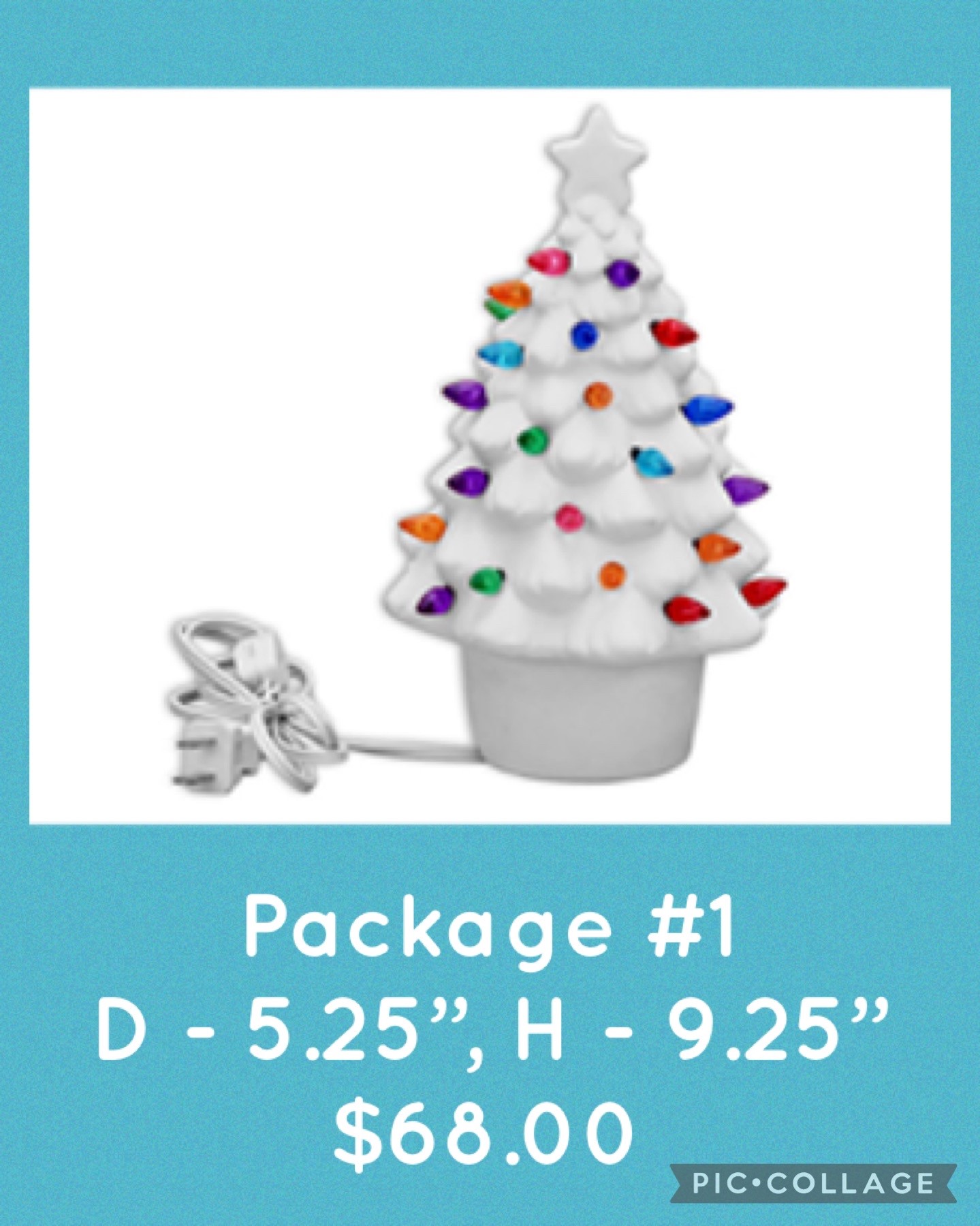This image features a picture collage with a light green border and a white background. At its center is a white Christmas tree adorned with a white star on top, and white elements including the cord, plug, and base. The only non-white features on the tree are the multicolored lights, which come in purple, green, orange, red, and blue. "Package number one" is texted alongside dimensions "D-5.25, H-9.25" and a price of $68. A bottom banner indicates this is a "pic collage." The overall design leaves some ambiguity, suggesting the tree could be a tree topper, a decorative light, or a table ornament.